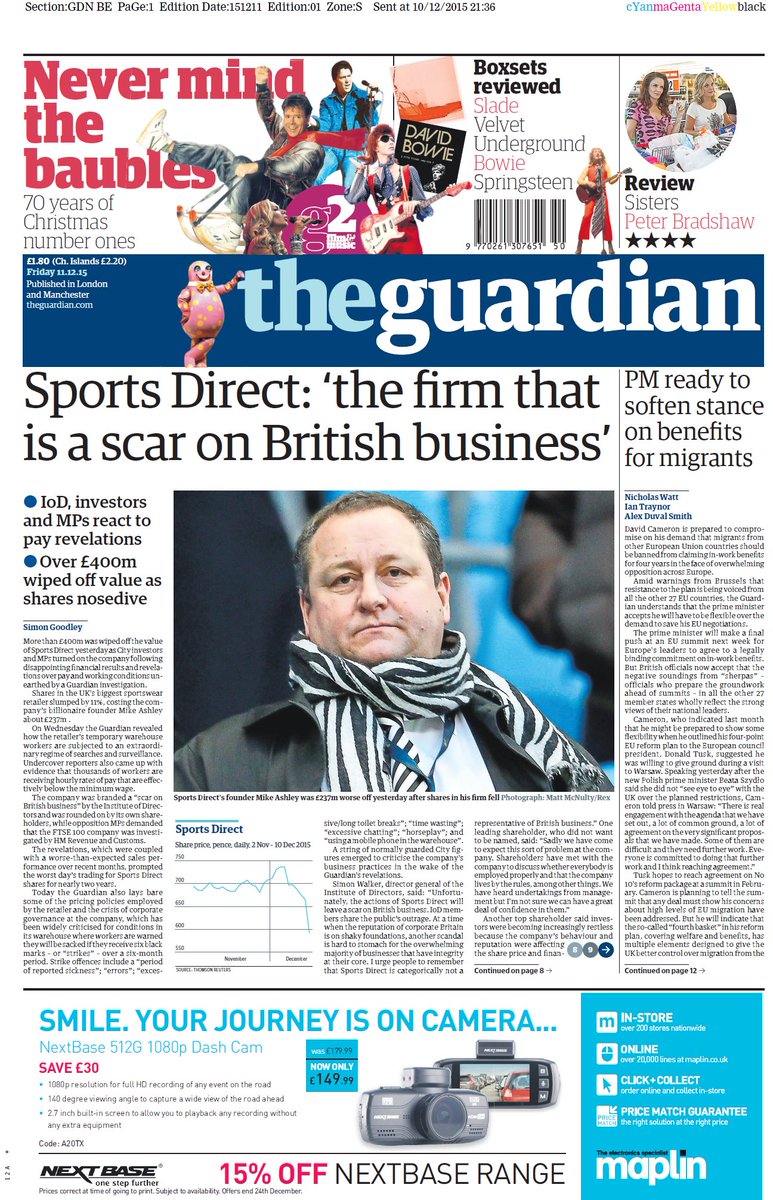This is a screenshot of the front page of The Guardian, a prominent British newspaper. The main feature of the page is a headline article titled "Sports Direct: The Firm that is a Scar on British Businesses." Accompanying the article is a photo of a white male wearing a scarf, although the caption identifying him is too small to be legible. To the right of the main article, there are additional headlines, including one titled "PM Ready to Soften Stance on Benefits for Migrants." At the bottom of the page, there are several advertisements promoting a camera.